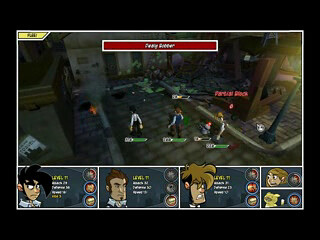This is a screenshot from a video game likely played on a computer. The image itself is small and depicts three or four characters walking along a stone sidewalk. The viewpoint is from behind the characters, showing their backs as they move towards a building in the background. The scene is festive, with confetti or similar effects filling the air. At the bottom of the screen, there are cartoon avatars accompanied by small text paragraphs, presumably displaying the characters’ names and some information, although the details are too tiny to discern.